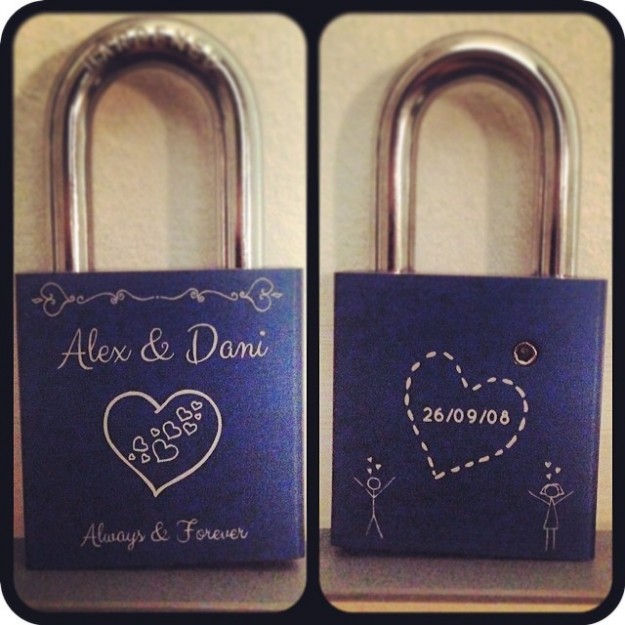This image, with a black border and beveled corners, features two photographs of a single blue metallic padlock with a goldish brass loop, set against a yellowish beige background. The photograph on the left side depicts the front of the padlock. Inscribed in elegant calligraphy are the names "Alex & Dani," with a large heart beneath them containing approximately ten smaller hearts. Below this, the words "always & forever" are elegantly etched in a goldish tint, emphasizing a flourishing script.

The photograph on the right side shows the rear of the padlock, which features a dashed heart slightly tilted to the right. Within this heart, the date "26/09/08" is inscribed, suggesting September 26, 2008. At the bottom of this side, two stick figures are depicted: the left figure seems to be male, characterized by its simplistic design and three hearts above its head; the right figure appears female, denoted by a V-shaped dress and hair, with arms outstretched and three hearts above its head, resembling signs of affection.

These visual elements collectively symbolize the deep devotion and enduring love between Alex and Dani.